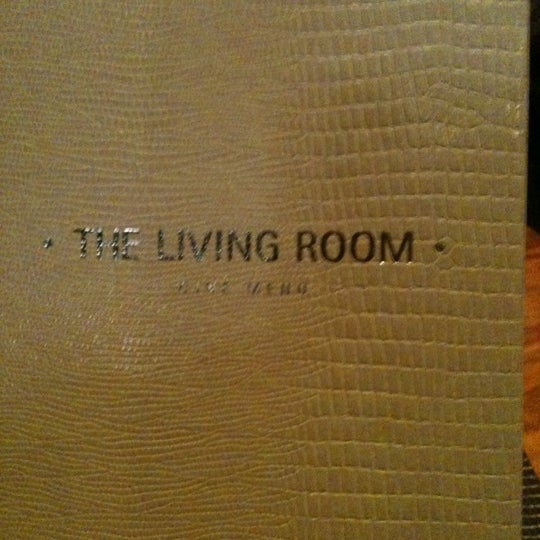The image primarily features a yellow diary cover that dominates the frame, leaving only a small portion on the right side uncovered. The diary has "THE LIVING ROOM" written prominently in capital black letters in the middle of the image. Below these words, there's another line that appears blurred and difficult to read, possibly consisting of two short words around four characters each. The cover exhibits various patterns, including horizontal, wavy, and square designs, which suggest a textured appearance that could resemble leather or animal skin, possibly snake skin. The texture features smaller squares on the left side that become larger and less dense towards the right.